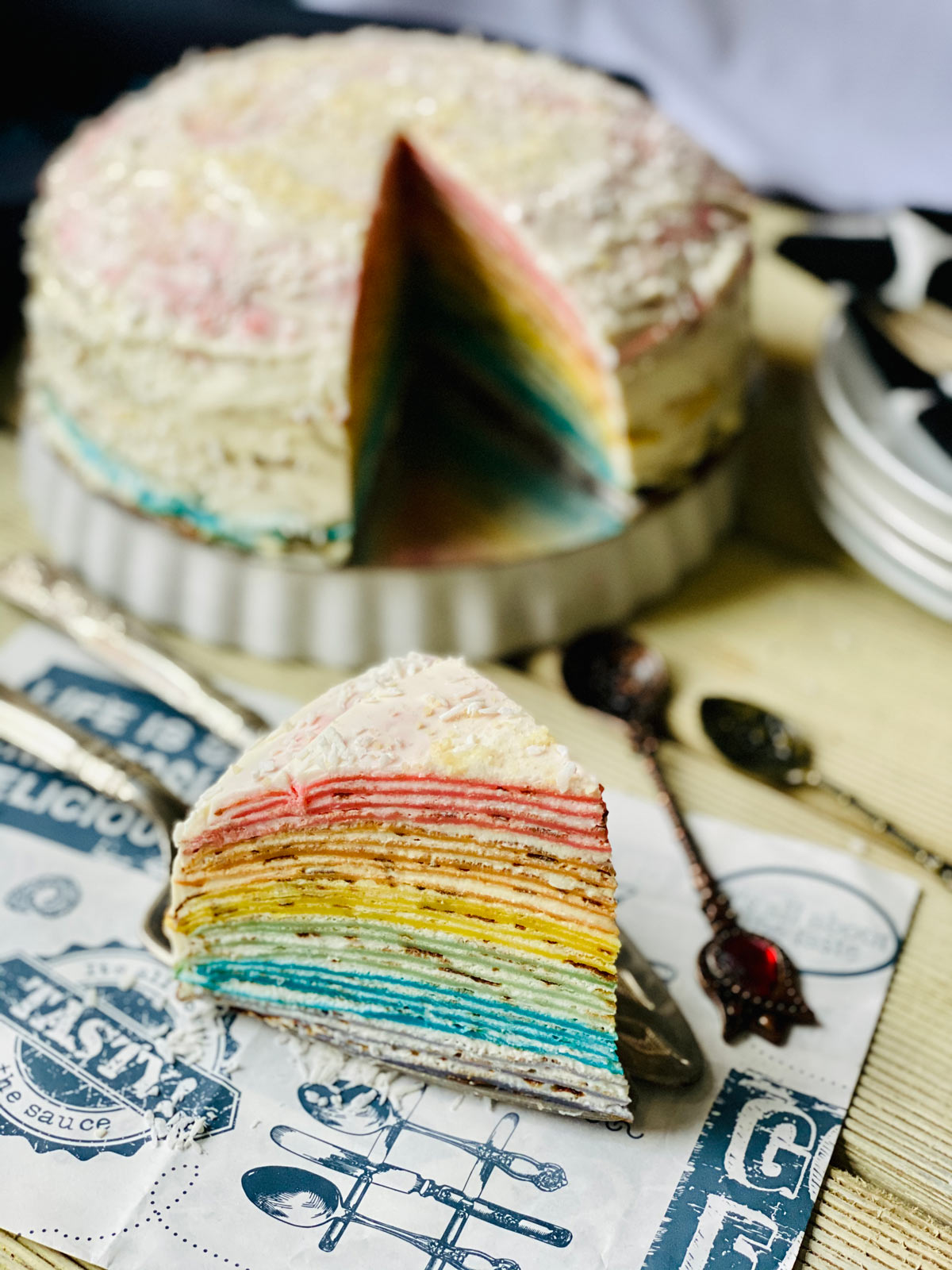The image features a meticulously detailed slice of rainbow cake placed on a printed decorative napkin that is emblazoned with images of silverware and the word "tasty." The cake slice, centrally positioned in the lower part of the image, reveals its strikingly thin layers of vibrant colors: a mix of red or pink at the top, followed by yellow, light green, green, blue, and a brighter blue. The outer layer of the cake is adorned with white icing, which appears slightly blurred towards the back, blending with the rest of the cake that occupies the upper back portion of the photo. The even and neat layering of the cake is visible where it has been cut. A pie slicer supports the slice, resting on a wooden table. To the right of the main cake, partially visible, is a tidy stack of plates alongside two neat spoons extending back towards the cake plate, harmonizing with the professional and carefully arranged aesthetic of the photograph.